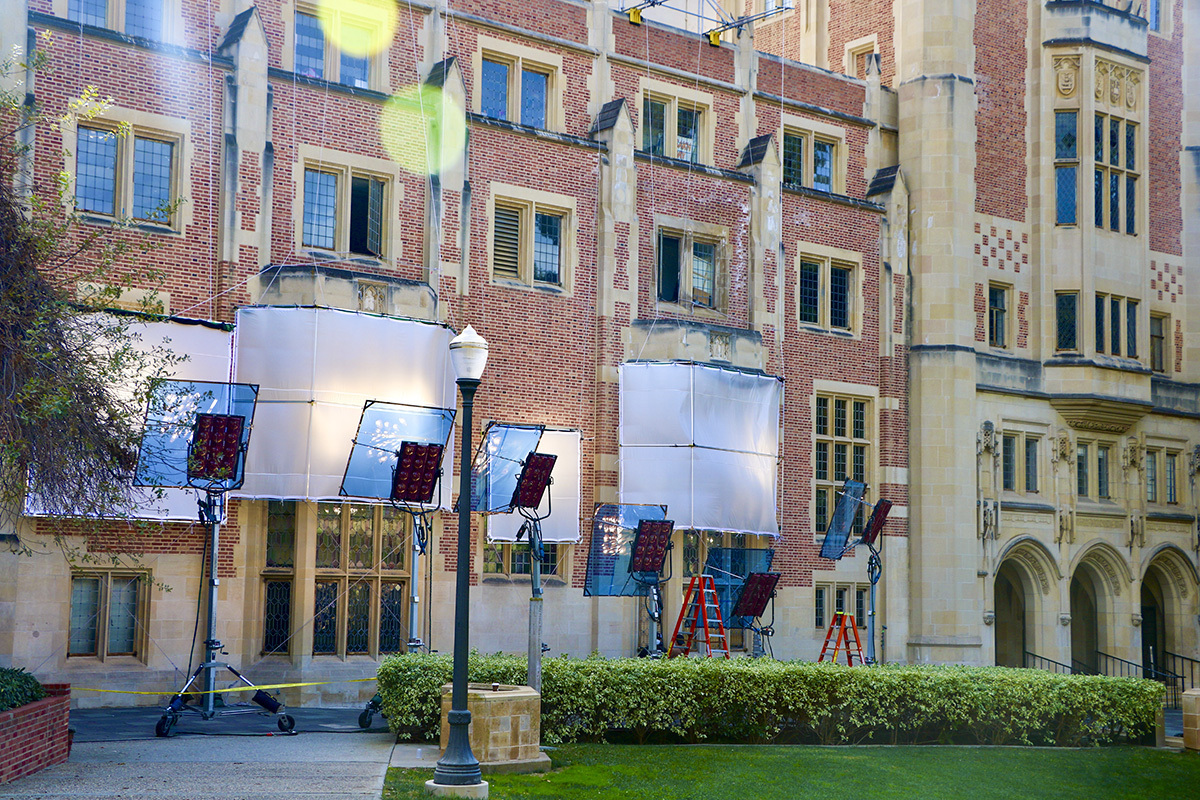The image depicts an old brick building reminiscent of Victorian or English architecture, possibly an apartment building, school, or even a film set designed to look like such an institution. The red brick structure is accented with tan detailing around the numerous windows, and features distinct architectural elements including archways and steps. The presence of a hedge and lampposts in front amidst green grass further accentuates its classic educational institution vibe, hinting at an Ivy League school or prestigious university setting. Various studio lights and blue screens set up around the building suggest that it is currently being used as a movie or TV set. The lights project through the windows, illuminating the building's interior, with additional equipment like ladders visible, indicating an active filming scene.